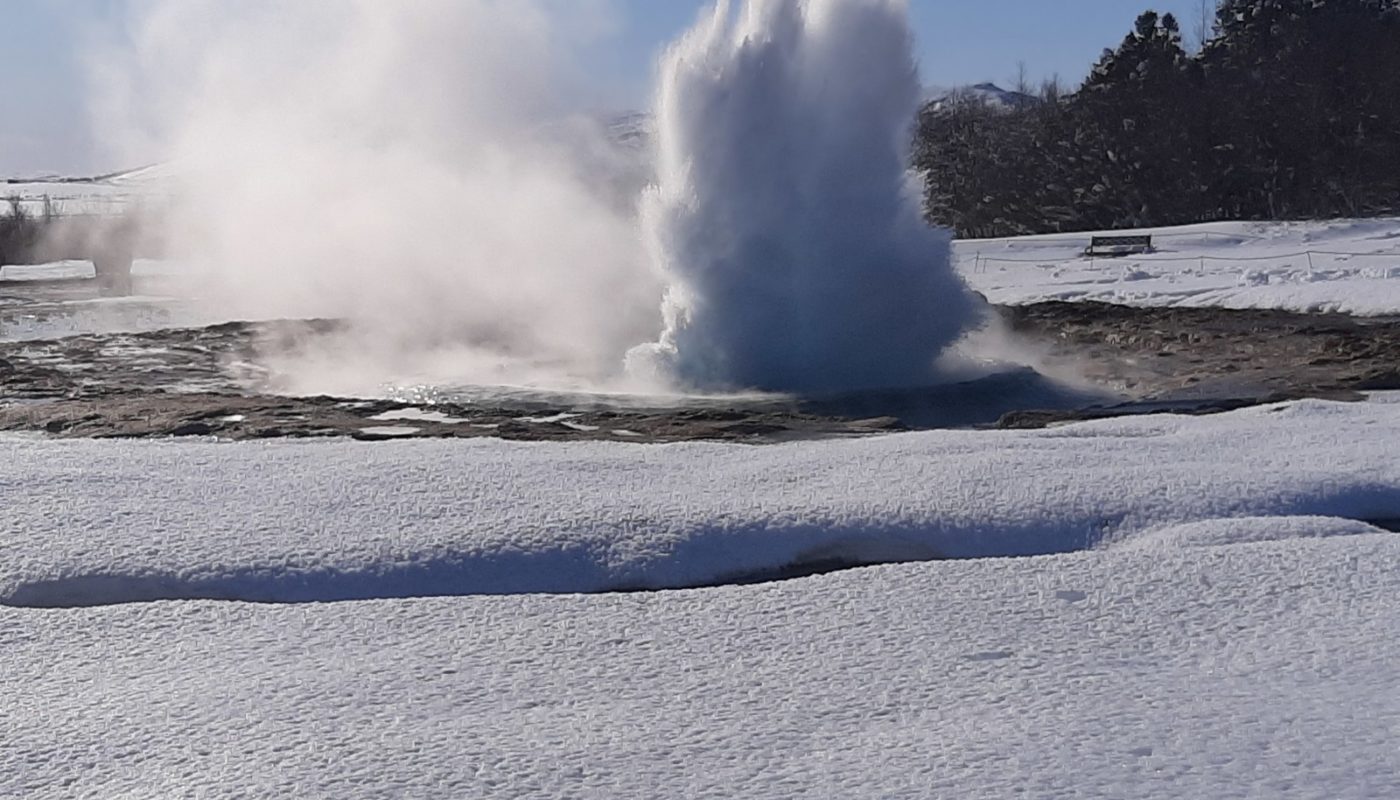The photograph captures a breathtaking scene of nature centered around an erupting geyser. Positioned almost perfectly in the middle of the image, the geyser shoots out a dramatic column of sparkling water and billowing steam, reminiscent of an explosive burst of snowy brilliance. Encircling the base of the geyser is a dark grey, crater-like structure, which provides a stark contrast to the snowy ground surrounding it. This snow, rough in texture, blankets the scene, lending the photo a predominantly white hue. To the right, a cluster of dark green pine trees brings a touch of color and further contrast against the snow and steam. A bench-like structure is subtly visible in the top corner, suggesting a spot for visitors to admire this natural wonder. Above, the sky stretches out in a clear, perfect blue, framing the misty plume that rises from the geyser and enhancing the image’s serene yet powerful ambiance.